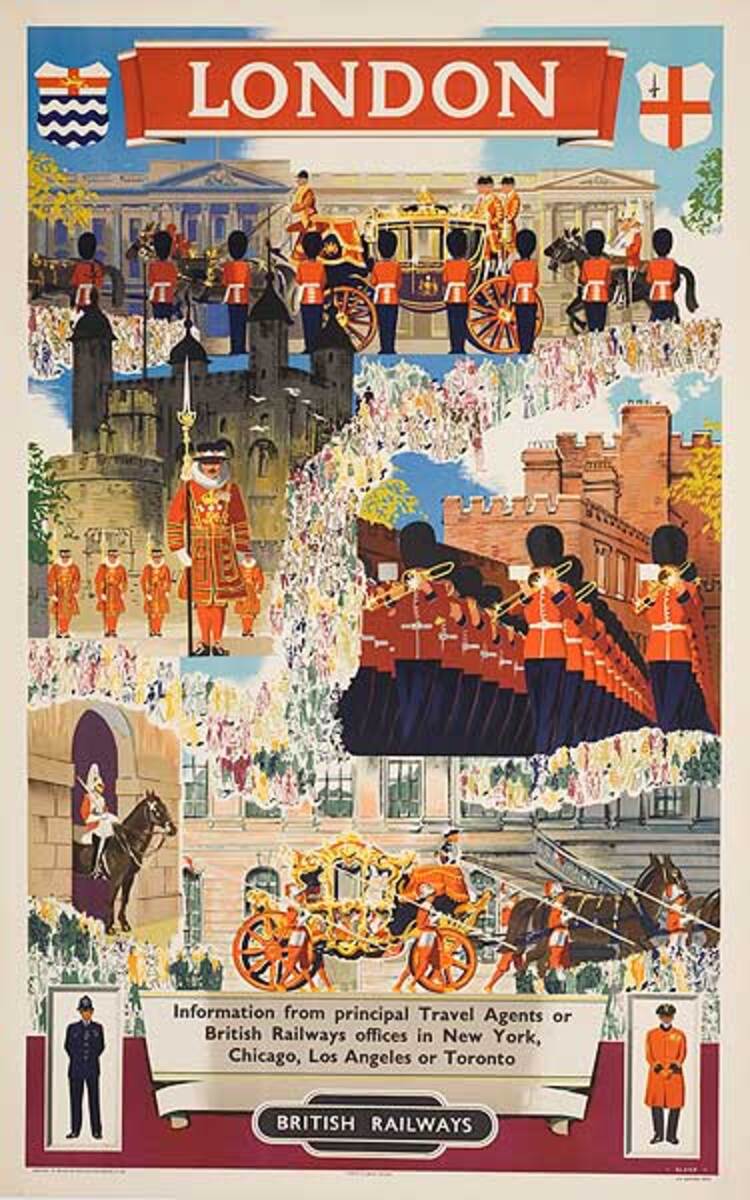This advertisement for British Railways, likely a scan of an old poster, boasts a vibrant, cartoon-like drawing that meticulously captures iconic British scenes. Topping the poster, a red ribbon banner inscribed with "London" in white letters immediately draws attention. One of the focal figures is the Royal Guard, clad in the distinctive red suit and wielding a spear-like weapon, stationed in front of an imposing castle, reminiscent of Buckingham Palace.

The central section enriches the narrative with hand-drawn artwork of the British military band, depicted in red and black uniforms, playing horns in a ceremonial display. Also included is an elaborate gold carriage, escorted by guards, providing a glimpse into British pageantry.

The lower part of the poster features a detailed image of a horse-drawn carriage, artistically rendered, showcasing the grandeur of a city scene. Supporting these visuals, informative text advises that further information can be obtained from principal travel agents or British Railways offices in New York, Chicago, Los Angeles, and Toronto. This is reiterated with the bold "British Railways" tag at the bottom, rounding out a compelling and comprehensive visual journey through Britain's cultural heritage.